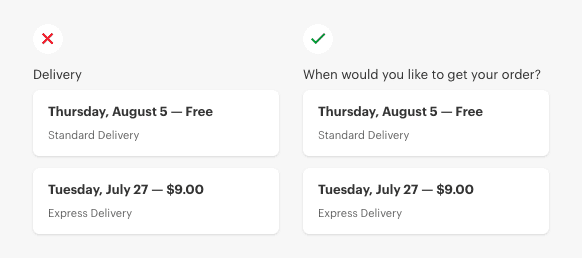This image depicts a delivery options page on a website. In the top left corner, there is a white circle with a red 'X' icon. Below this, the word "Delivery" is displayed in black text. Moving further down, there is a white box containing the text "Thursday, August 5th - Free" in bold black letters, followed by "Standard delivery" in gray letters.

Further down on the left side, another white rectangular box contains the text "Tuesday, July 27th - $9" in bold black letters, with "Express delivery" in gray letters below it.

In the top right section of the image, there is a green circle with a white checkmark. Directly below, it says "When would you like to get your order?" in gray text. Further down, there is another white rectangle with the text "Thursday, August 5th - Free" in bold black letters and "Standard delivery" in gray letters below. Below this rectangle, there is an additional white rectangle that has "Tuesday, July 27th - $9" in bold black letters, followed by "Express delivery" in gray letters.